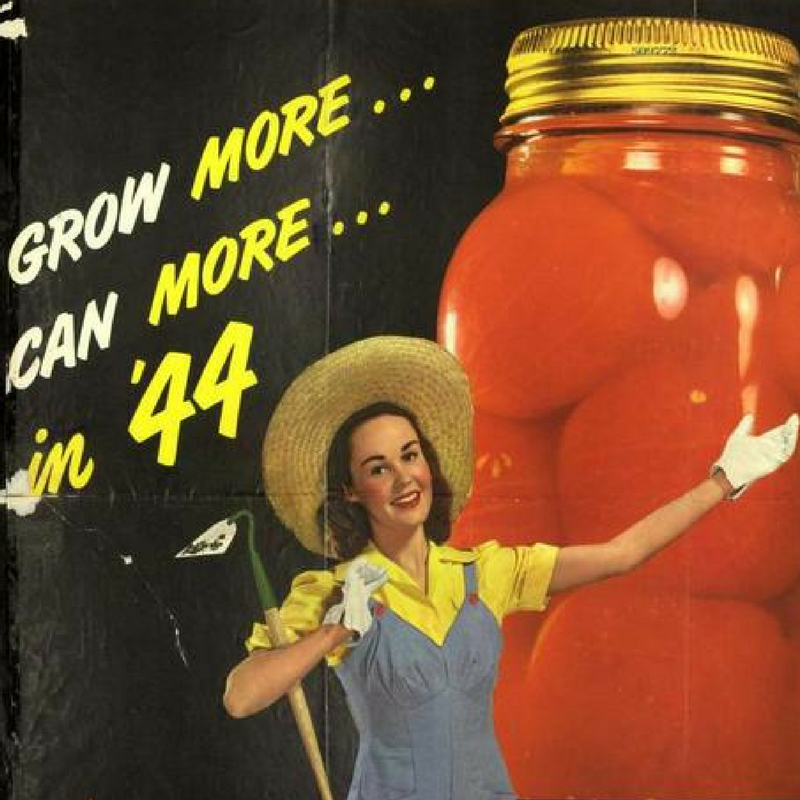In this vintage ad, likely torn from a magazine, we see a vibrant and detailed graphic image featuring a smiling young woman in her mid-20s. She stands in the lower center of the poster, wearing a wide-brimmed straw hat, a yellow T-shirt under a blue pinafore dress, and white gloves. Her left arm is raised in the air while her right arm is wrapped around the handle of a shovel or garden hoe, which has dirt on its tip and features brown and green tones along the handle. The background prominently showcases a tall, large glass jar filled with whole tomatoes, extending from the upper right to the center of the image, with a gold twist cap. Positioned in the upper left corner, bold yellow text reads "grow more, can more in '44," with the words "grow" and "can" highlighted in white. Every intricate detail of the design contributes to the ad's vintage charm and its message promoting gardening and canning during 1944.